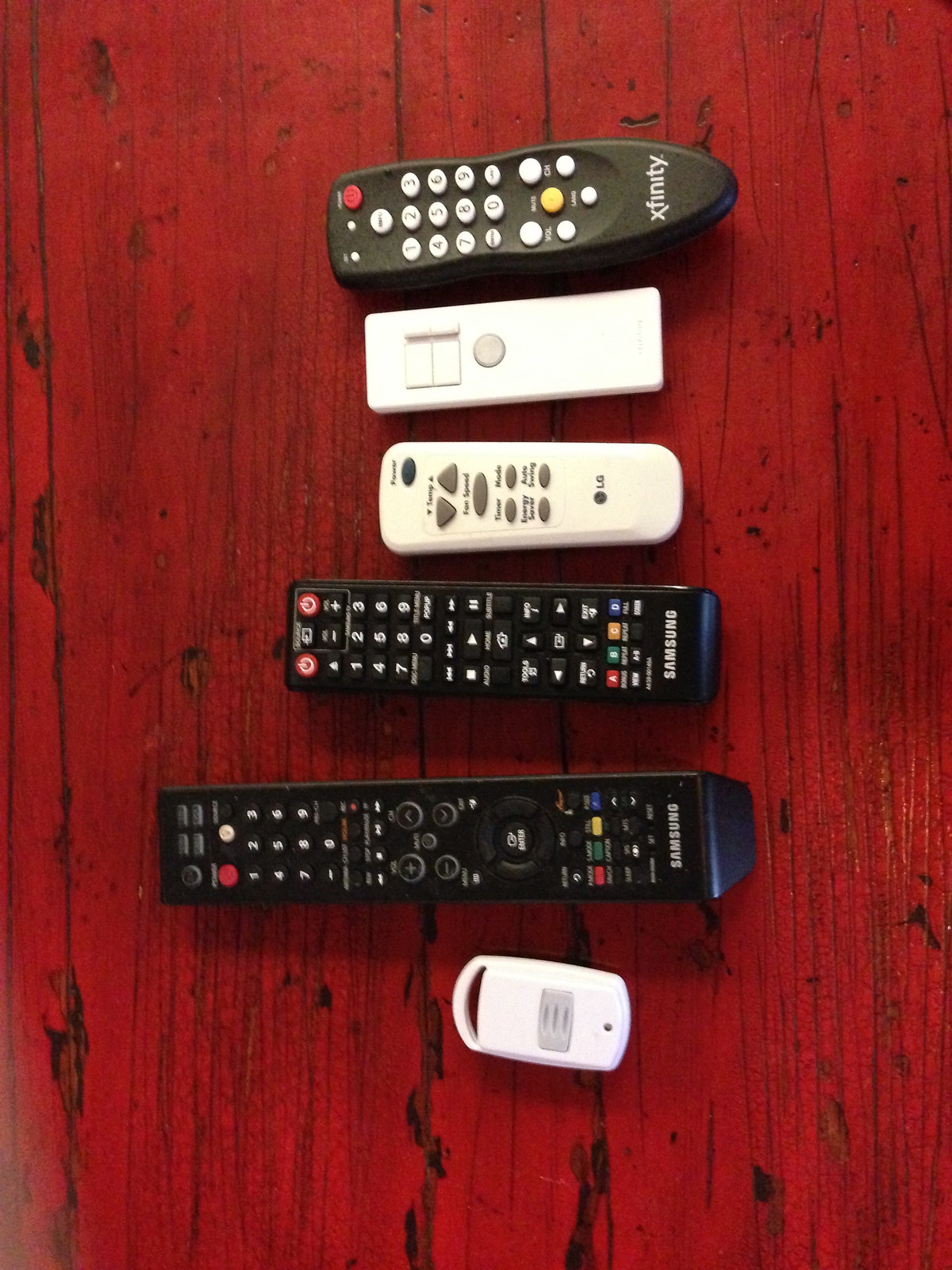In the image, we're looking straight down at a Cherrywood table adorned with six remote controls. The reddish hue of the Cherrywood serves as a warm backdrop to this assortment of remotes. Three of these remotes are black and three are white. The black remotes include two from Samsung with distinct features: one is shorter with numerous black buttons highlighted in white, and the other is longer with a central circular pad for navigating and red, green, yellow, and blue buttons along the bottom. The third black remote is for Xfinity, marked by its distinctive white keys, a yellow button in the middle, and a red button on the top right.

The white remotes include one for an LG fan, easily identified by its numerous gray buttons in a triangular layout. Another white remote is small, square, with a single button in the center, evoking the design of an emergency alert device. The final white remote, also minimalistic, features a singular central button, likely used for a straightforward task such as garage door functionality. All six remotes are carefully arranged in the center of the table, painting a picture of a multifaceted entertainment setup.